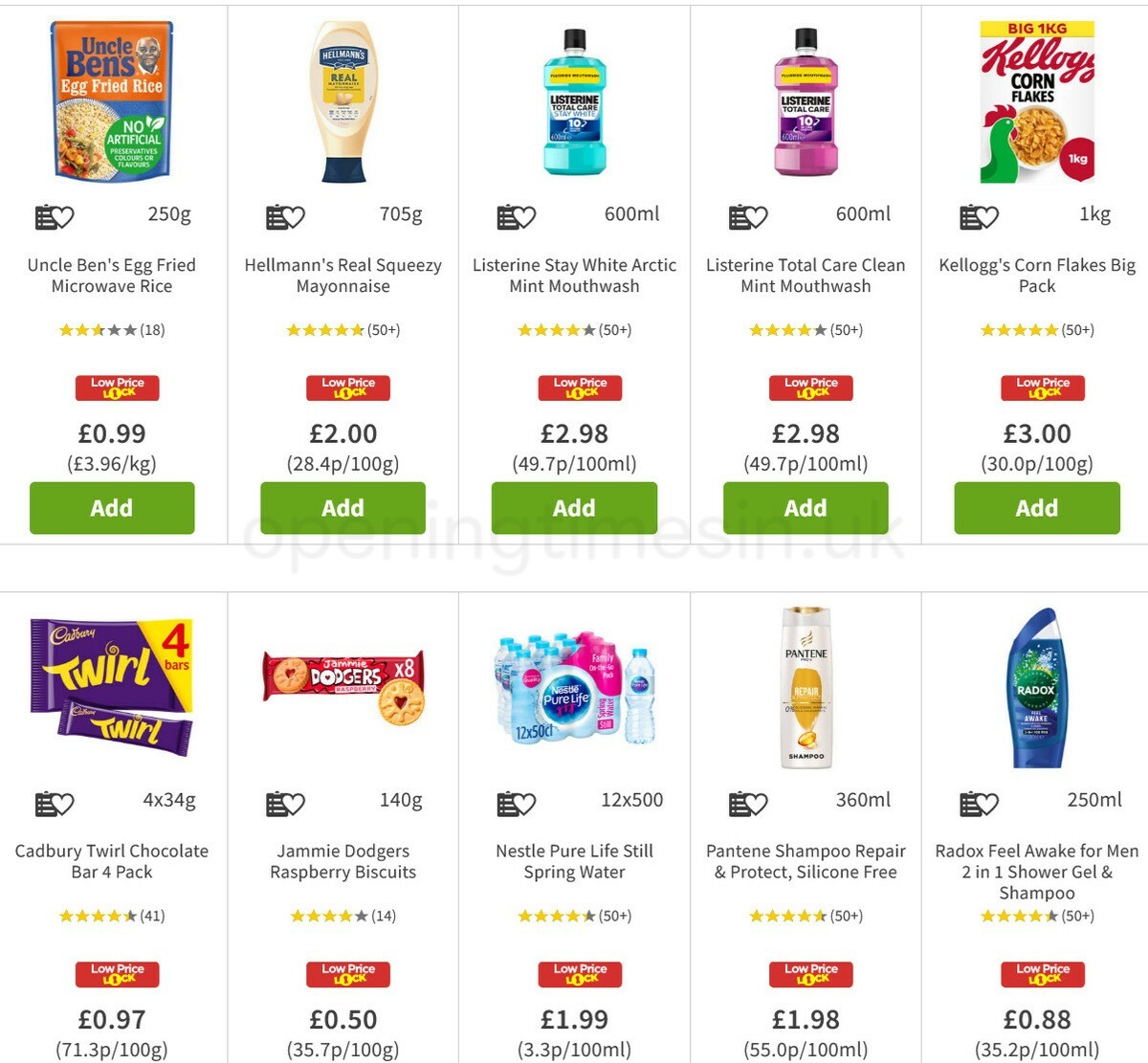The image depicts an assortment of grocery items available for online purchase, each priced in pounds, suggesting the location may be a country like Australia. The items are organized in two rows, each featuring five distinct products. 

Starting from the top row:
1. Uncle Ben's Basmati Rice is priced at £0.99.
2. Hellman's Real Mayonnaise costs £2.00.
3. Listerine Stay White Arctic Mint Mouthwash is available for £2.98.

Each product listing includes several details:
- The product name and its price.
- A star rating out of five, indicating customer reviews.
- A "low price lock" feature, ensuring competitive pricing.
- An "Add to Cart" button for convenient shopping.

Additional products include:
- Listerine Total Care Clean Mint Mouthwash.
- Kellogg's Corn Flakes Big Pack.

The detailed setup ensures that shoppers can easily discern product information, prices, and review ratings, enhancing the online shopping experience.